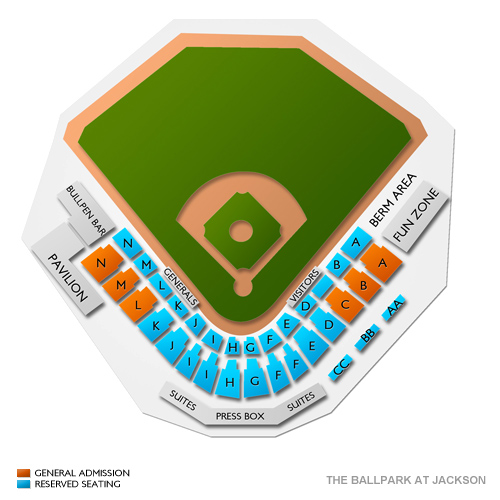This detailed graphic of a baseball field highlights several key features of the ballpark. The field itself is depicted with distinct green (grass) and brown (dirt) areas, surrounded by various seating and functional sections. The stands are showcased with blue and orange seats arranged in sections labeled with letters such as N, M, L, K, J, I, H, G, F, E, D, B, and A. The blue seats indicate reserved seating areas, while the orange sections, marked N, M, L, C, B, and A, are designated for general admission.

Additionally, the image includes various amenities within the ballpark, such as the Bullpen Bar and a pavilion. On top of the seating areas, there is a series of suites and a press box for special guests and media personnel, noted at the very top of the seating diagram.

Also featured are specific sections such as a berm area and a fun zone designed for family-friendly activities. Special sections marked C, C, B, B, and A, A are located higher up in the stadium.

The bottom corner of the graphic presents the name of the venue, "The Ballpark at Jackson," set against a mostly white background with a sunny ambiance. The image is filled with vibrant colors including blue, orange, and green, enhancing the viewer’s understanding of the ballpark’s layout and seating options.